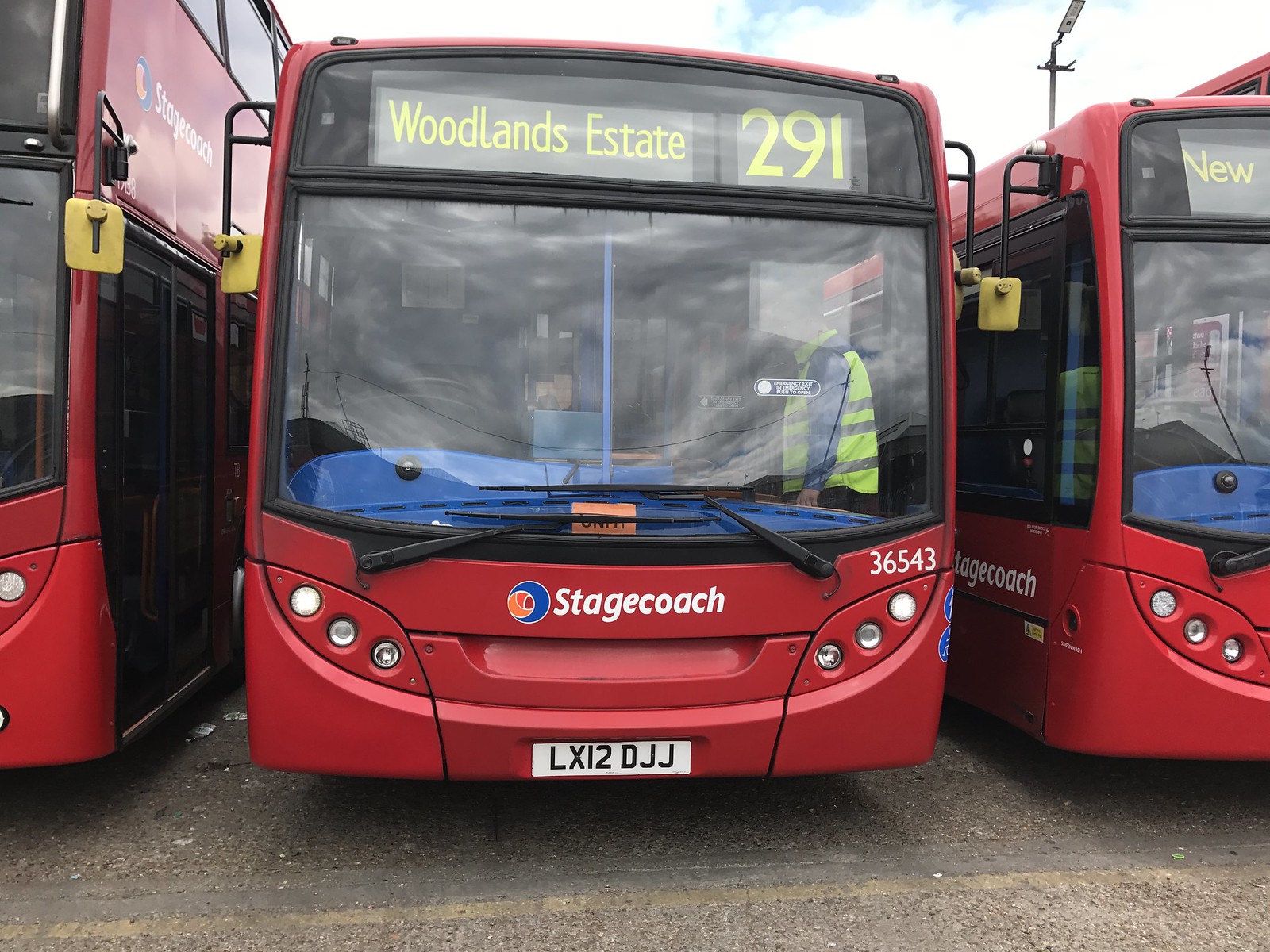The image captures an outdoor scene with three parked red buses, viewed from the front. Dominating the center is a single-deck bus marked with "Woodlands Estate 291" at the top of its large front window. The bus prominently displays "Stagecoach 36543" across its front, accompanied by a license plate reading LX12DJJ and three lights on each side at the bottom. Inside, just behind the door, stands a man dressed in a high-visibility safety vest and a blue or gray shirt. Flanking this central bus, a red double-decker bus is visible on the left. Only its front-right section and upper deck can be seen, showcasing the word "Stagecoach" in white lettering atop. To the right of the central bus, another identical single-deck bus stands aligned. Though we can only partially view this bus from the side, it features "Stagecoach" and the partially visible word "new" at the top. The buses are situated on a concrete parking lot.